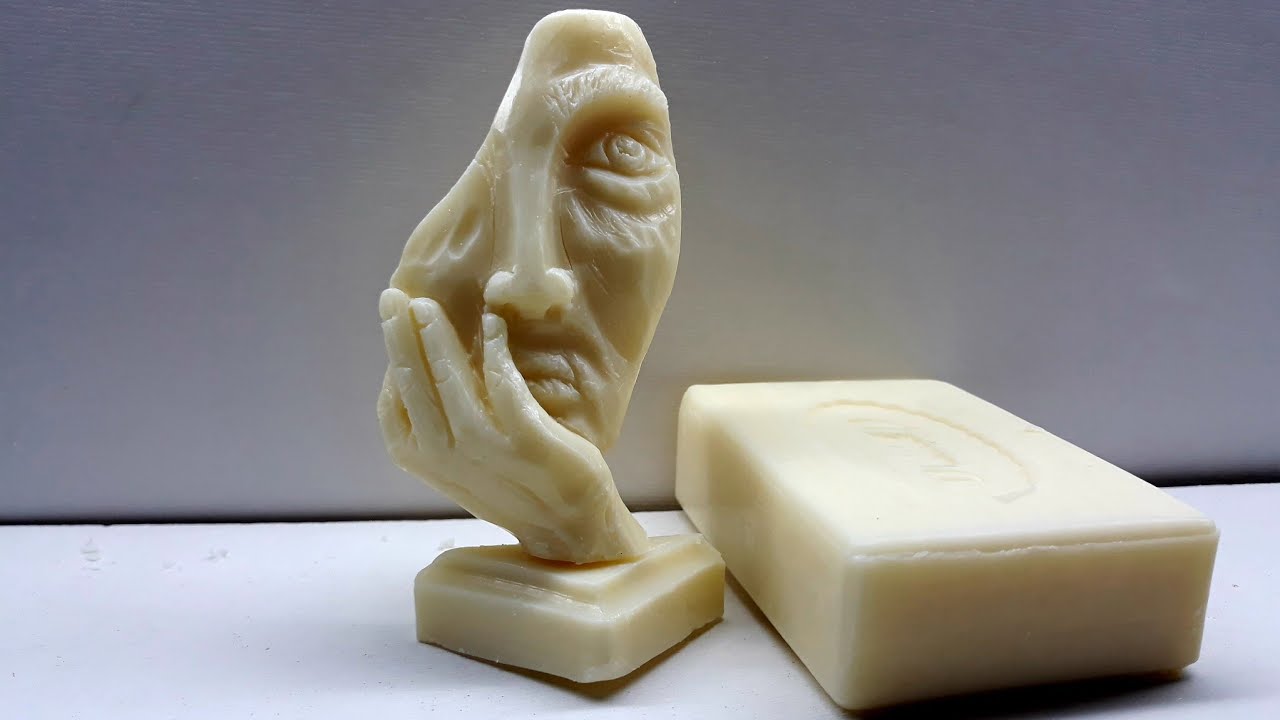The image showcases an intricate soap sculpture. On the right side, there's an untouched, rectangular bar of soap. To the left, the soap has been meticulously carved into a partial bust of a face, resting its chin on a detailed hand emerging from a triangular base with rounded, beveled edges. The sculpture's face is missing the left half, giving the impression of it melting away. The remaining features include a prominently detailed eye with a bag underneath, a defined eyebrow, and a sharp nose. The mouth area hints at the intention of a mustache, with a groove in the soap suggesting it. The hand cradling the face is remarkably lifelike, showing defined knuckles, fingernails, and visible bones. The sculpture exhibits an exceptional level of detail, showcasing the artist's skill in portraying lifelike features in an unconventional medium.